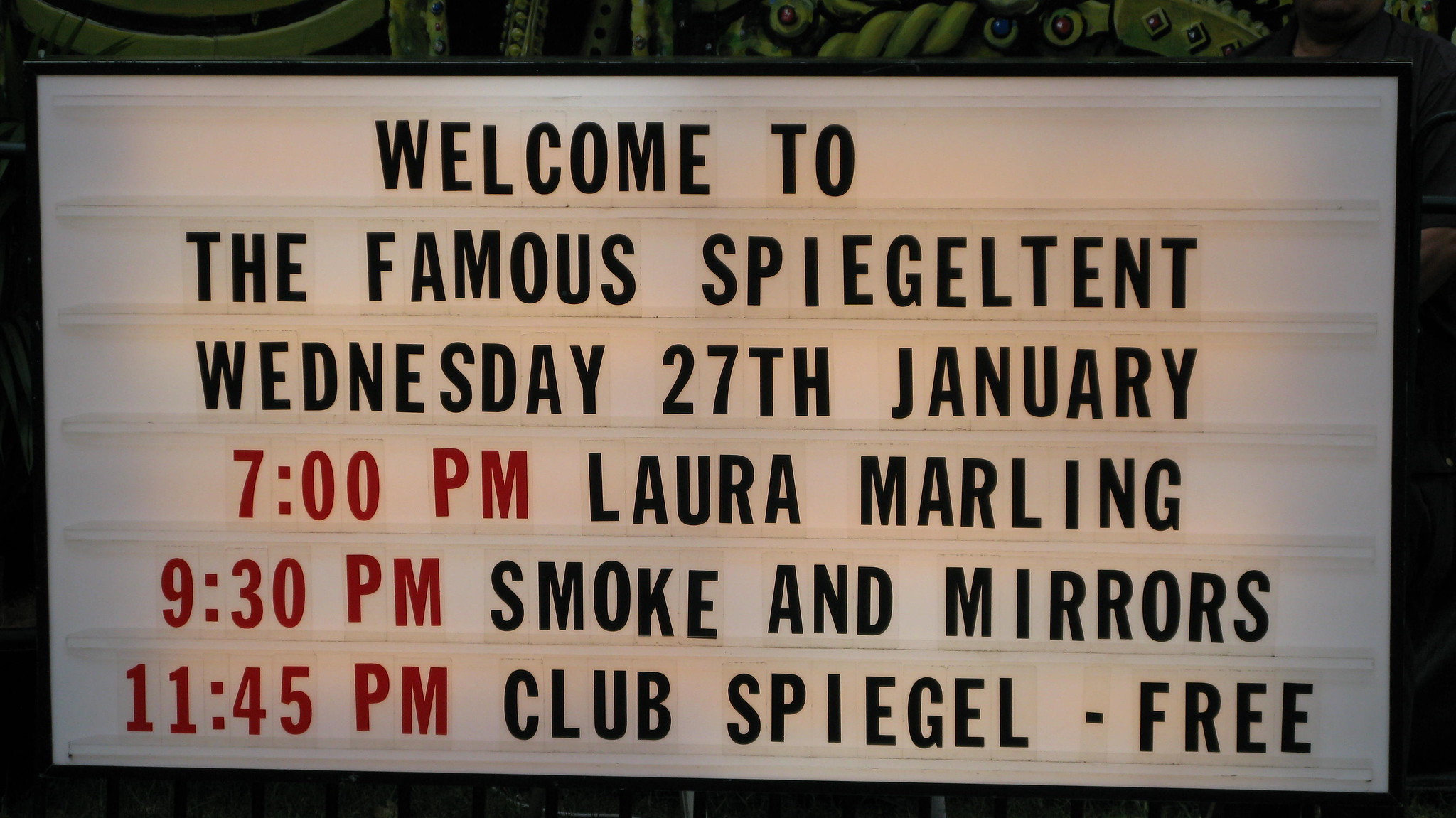Sign for a free concert at the renowned Spiegel tent featuring Laura Marlin's "Smoke and Mirrors" tour. The sign, designed in striking black and red lettering, lists the performance times: 7:00 PM, 9:30 PM, and 11:45 PM. The backdrop of the signage offers a glimpse of the beautiful day, enhancing the anticipation for the event. Join us at Club Spiegel for an unforgettable musical experience!